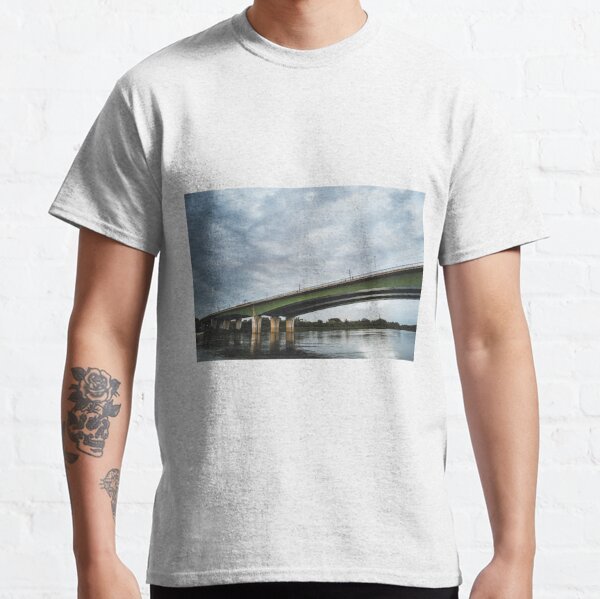The photograph captures the torso of a white-skinned man wearing a white t-shirt, seen from neck to waist. The t-shirt features a rectangular image centered in the front, depicting a straight green bridge with three supporting columns, spanning diagonally from the bottom left corner to the middle right against a backdrop of blue sky and clouds. The man has a detailed flower tattoo on his right forearm, visible on the left side of the image. The setting also includes a vague white brick wall in the background, and his pants, implied to be black, are only partially visible at the bottom of the frame.